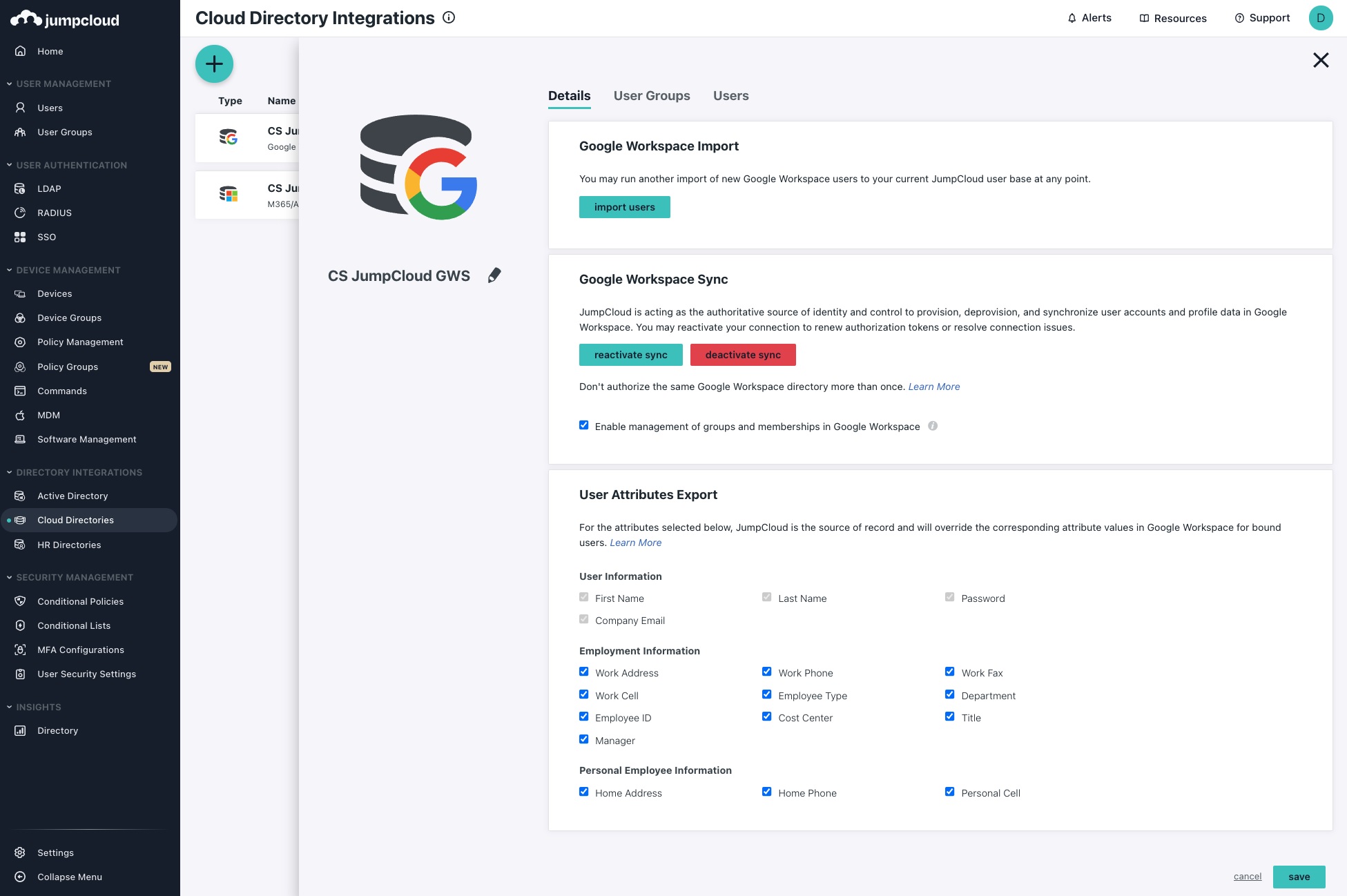The image depicts a computer screen showcasing the cloud directory integrations interface. At the forefront, a menu titled "Details" is prominently open, with "Details" highlighted in a darker shade, suggesting it has been selected from several options, including "User Groups" and "Users." Specifically, the page displays information related to a "Google Workspace Import."

On the left, a letter "G," emblematic of Google, is visible, accompanied by an icon resembling a canister behind it. Adjacent to this, the text reads "CS JumpCloud GWS," with a pencil icon next to it, perhaps indicating the option to edit. Centrally positioned is the "Google Workspace Sync," indicating the synchronization process with Google services. 

Towards the bottom, the section "User Attributes Export" is noted, featuring numerous attributes that users can selectively check or uncheck to customize their export preferences. On the left-hand side of the screen, a comprehensive navigation pane is visible, listing options such as "Home," "Users," "Users Guide," "Groups," "LDAP," "Radius," "SSO," and more. This menu extends downwards, culminating in sections labeled "Directory," "Settings," and an expandable "Collapse Menu" option, ensuring that users can manage their directory integrations thoroughly.